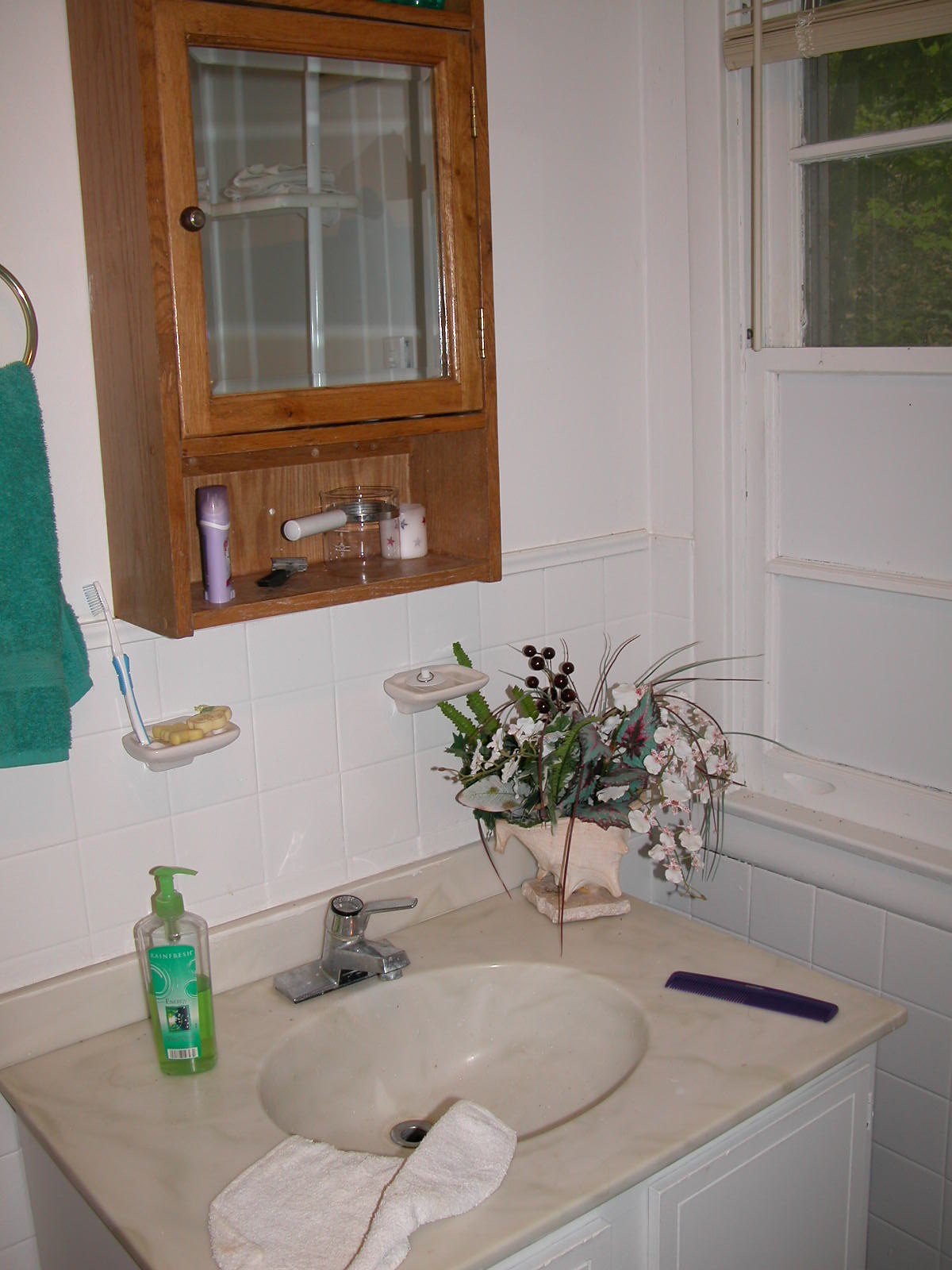This photograph captures a stylishly organized bathroom from the vantage point of the sink. The sink itself boasts a beige marble finish with white drawers beneath, presenting a clean and polished look. Atop the sink's countertop lie several essential items: a black comb, a neatly folded white hand towel, a soap dispenser filled with green liquid, and a charming floral arrangement, adding a touch of natural elegance.

Against the wall, two small pink-beige shelves are mounted. One shelf holds a white and blue toothpaste, prominently displayed for easy access. Above these shelves, a brown wooden medicine cabinet houses a collection of personal items, including deodorant, a brush, and a candle, bringing both functionality and a cozy ambiance to the space.

To the left of the sink, a silver hook supports a blue hand towel, ready for use. The upper right corner of the image highlights a window, inviting natural light into the room and offering a glimpse of the exterior, which adds a refreshing element to this well-appointed bathroom scene.